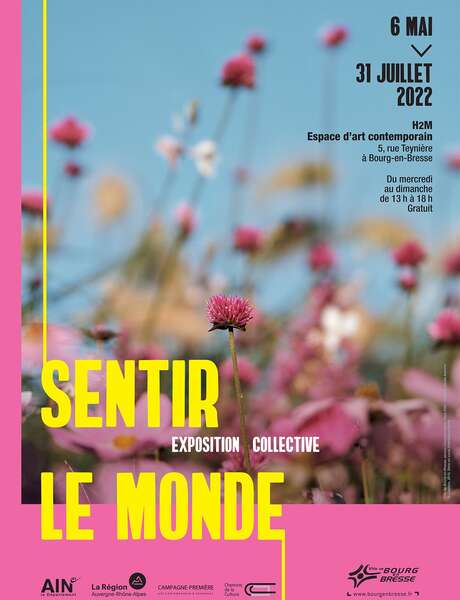The image is a detailed flyer for a French art show titled "Cintur Limonde", prominently displayed in solid yellow text. The event runs from May 6th to July 31st, 2022. The background features an array of pink flyers against a clear blue sky, enhancing the artistic appeal of the poster. The flyer is framed by a pink border that transitions from the bottom to the top left corner. 

Additionally, there is white text between "Cintur" and "Limonde" stating "Exposition Collective," emphasizing the collaborative nature of the exhibition. A black text blurb in the top right corner is also present, though it is not in English.

The logos of sponsors—AIN, La Region, Campagne Premiere, and another, smaller, unreadable one—are situated at the bottom of the flyer in solid black text. The main colors used in the flyer are yellow, white, and black, harmonizing with the pink flyers and the blue sky background. The overall aesthetic is completed by a single in-focus flower with pink petals, standing out amidst the blurred floral background.